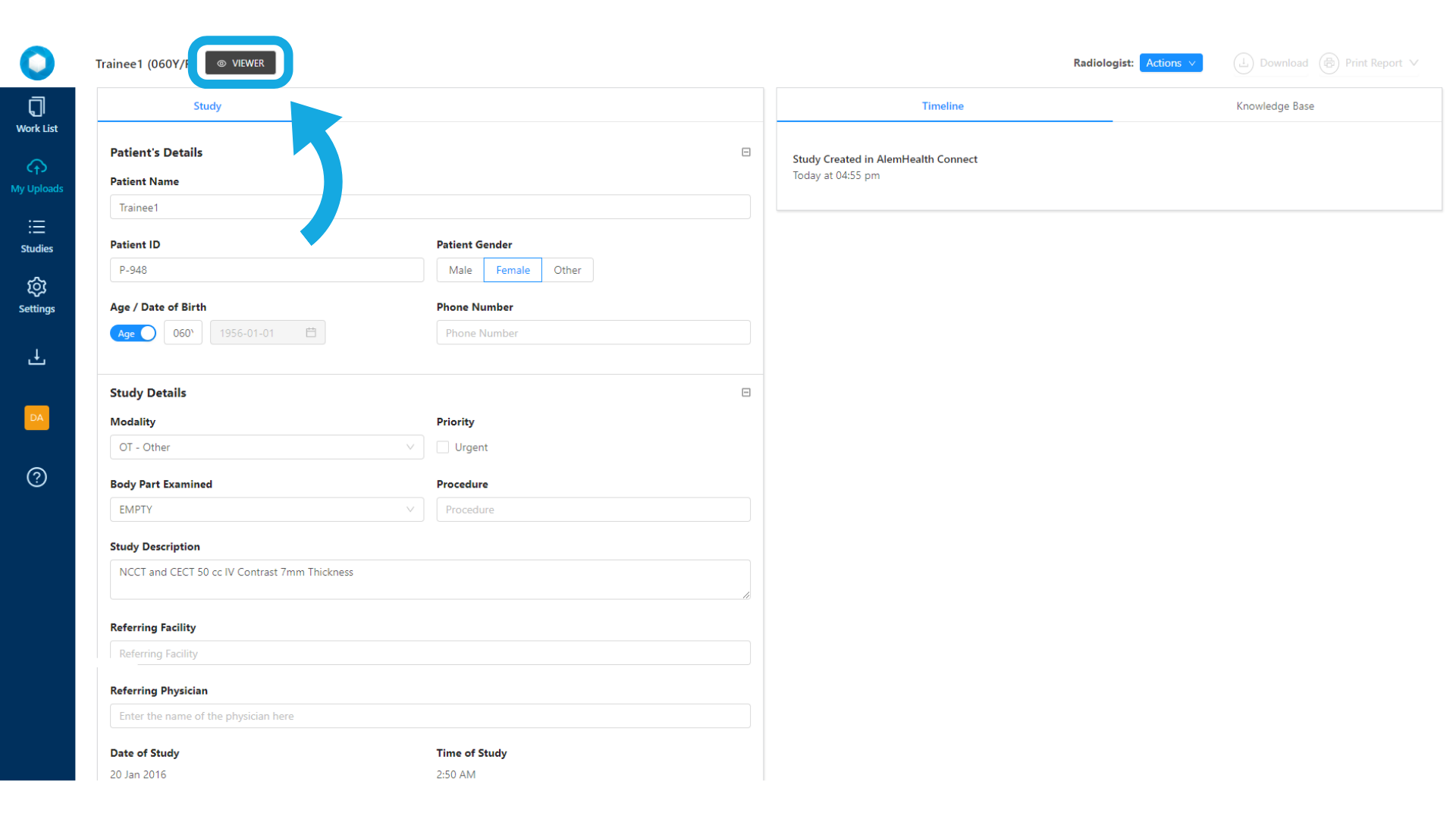In this image, we observe a software interface displaying various patient details and study information. The page features several text fields and categories, including a work list, my uploads, and studies. Detailed patient information is provided, such as:

- **Patient Name**: 21
- **Patient ID**: P-948
- **Age**: Born on January 1, 1956
- **Gender**: Female
- **Phone Number**: (Field is empty)
- **Modality**: OT (Other)
- **Body Part Examined**: (Field is empty)
- **Referring Facility**: (Not specified)
- **Referring Physician**: (Not specified)
- **Date of Study**: January 20, 2016
- **Time of Study**: 2:50 AM

The background of the interface is white, contributing to a clean and minimalistic appearance.